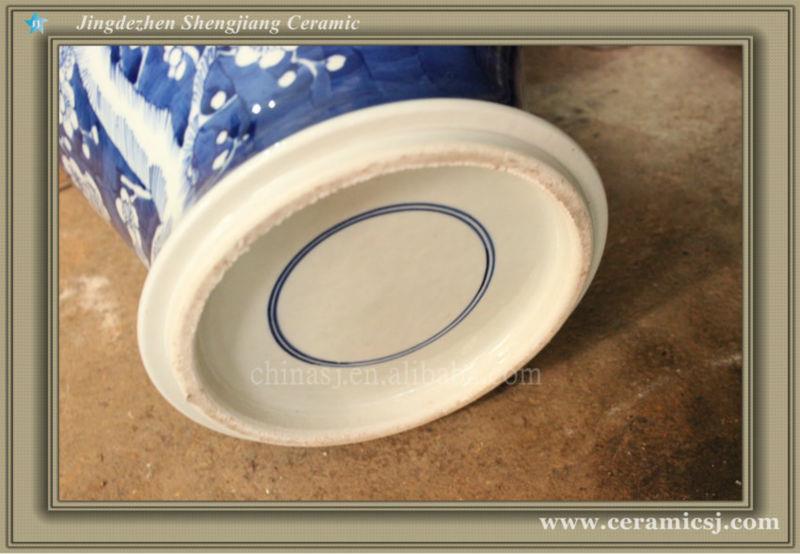The image is a detailed photograph of the bottom of a large ceramic pot, lying on its side on a gray cement floor. The pot, which appears to be made of fine China, features a rich blue and white design typical of chinoiserie, likely showcasing intricate patterns such as flowers or trees. The bottom of the pot is cream-colored, embellished with two concentric blue circles, forming a distinct ring.

The photograph is presented within a digital tan-colored border that mimics the appearance of a picture frame. At the top of this frame, white text reads "Jingdezhen Shengjiang Ceramic." In the bottom right corner, it reads "www.ceramicsj.com." Additionally, a watermark runs across the center of the photograph, indicating "Chinasj.en.alibaba.com," hinting at its origins and potential authenticity from Jingdezhen, a renowned center for Chinese ceramics.